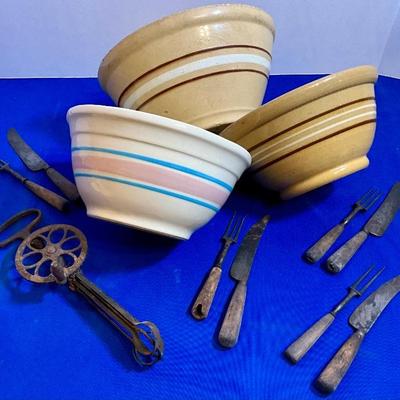The photograph features three ceramic pottery bowls artistically arranged on their sides, forming a triangular formation against a vibrant, bright blue table. Two of the bowls, which appear to be part of a set, are beige-brown with dark brown and white stripes, exhibiting identical tops and bottoms. The top and right bowls share this design. The third bowl, positioned on the lower left, differs by having a white background with a design of two thin blue stripes flanking a thicker pink stripe in the center. Alongside these visually striking bowls lie a collection of antiquated kitchen utensils, including three sets of tarnished, rustic forks and knives with wooden handles, and an old, hand-crank egg beater exhibiting signs of wear and distresses in the metal. An additional fork and knife set lies to the other side of the bowls. The settings and tools evoke a nostalgic, antique aesthetic, contrasting sharply with the luminous blue background that adds a modern vibrancy to the scene.